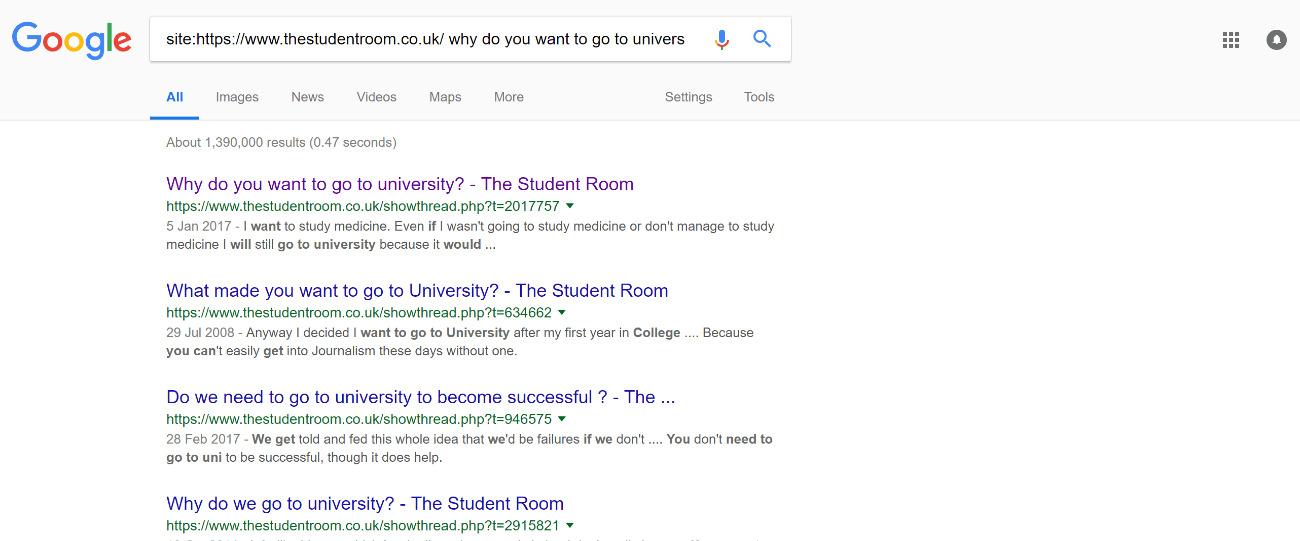This image appears to be a screenshot of a computer displaying a Google search results page. 

At the very top, there is a gray border with the word "Google" situated in the upper left corner. To the right of this, a white address bar shows the URL "thestudentroom.co.uk." Adjacent to the address bar, there are a microphone icon and a search icon. Below this section, several headings are displayed in a horizontal row: "All," "Images," "News," "Videos," "Maps," "More," "Settings," and "Tools." The "All" heading is underlined and highlighted in blue, indicating it is the selected category.

Beneath these headings, there is a small text noting that the search results number about 1,390,000 and were retrieved in 0.47 seconds. The page shows four main search results. 

1. The top result is displayed in purple and reads "Why do you want to go to university? - The Student Room." Its brief description states: "I want to study medicine. Even if I wasn't going to study medicine or don’t manage to study medicine, I will still go to university because it would..."

2. The second result has the title "What made you go to university? - The Student Room." Its description mentions: "Anyway, I decided I want to go to university after my first year in college because you can't easily get into journalism these days without one."

3. The third result is titled "Do you need to go to university to become successful?" Its description reads: "We get told and fed this whole idea that we'd be failures if we don't. You don't need to go to uni to be successful, though it does help."

4. The fourth and final result is "Why do we need to go to university? - The Student Room."

The layout is typical of a Google search results page, with specific focus on queries related to the necessity and reasons for attending university, all sourced from "The Student Room" website.